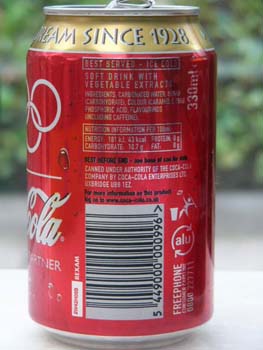The image showcases a white floor with a prominently placed can in the background. The can, though supposed to be green, is actually red and features gold accents. This particular can design dates back to 1928. On the left side of the can, the branding highlights Coca-Cola as an Olympic partner, displaying the Olympic rings. However, only two full rings and part of a third ring are visible in the image. Additionally, the can includes a message recommending that the drink is best served ice cold and mentions it is a soft drink with vegetable extract. The word "Coca-Cola" is repeatedly visible across the can. A barcode is situated to the right, and in the background appears to be what looks like a trash can and someone holding a stick or poking device. There is also a partially visible text that seems to say "free phone something."